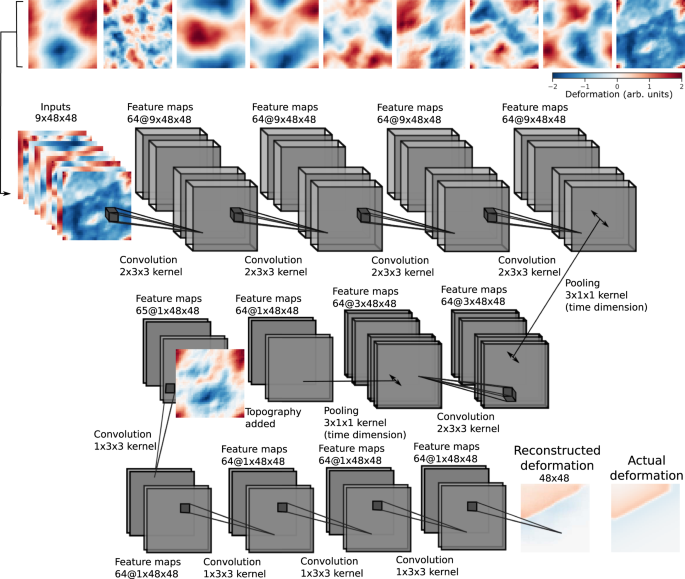The image is a detailed diagram featuring various stages of a graphical process. At the top of the diagram, there are nine distinct squares displaying splotches of red, blue, and white colors, with occasional black streaks, resembling a tie-dyed effect. These squares seem to represent different deformation states, as indicated by a nearby chart which maps these colors to numerical values: -2 is dark blue, -1 is medium blue, 0 is white, 1 is light red, and 2 is the darkest red.

Below these nine images, the right side hosts a detailed chart that aligns these colors with their respective numeric values. This section is labeled "deformation" and highlights how various hues represent different levels of deformation, spanning from dark blue (-2) to deep red (2).

Continuing down the diagram, the second row on the left shows additional squares with colorful splotches, while four adjacent rows comprising all-gray squares with interconnecting lines immediately follow. These gray squares feature dimensions and indicators above them, such as numbers, letters, and arrows.

Further below, subsequent rows predominantly contain gray squares. However, interspersed among them are colored squares similar to those at the top, indicating ongoing processing stages. Detailed labels, such as "inputs 9x48x48" and "feature maps, 64 at 9x48x48," specify the structure and size of these elements, with lines tying all components together to illustrate their relationships within the diagram.